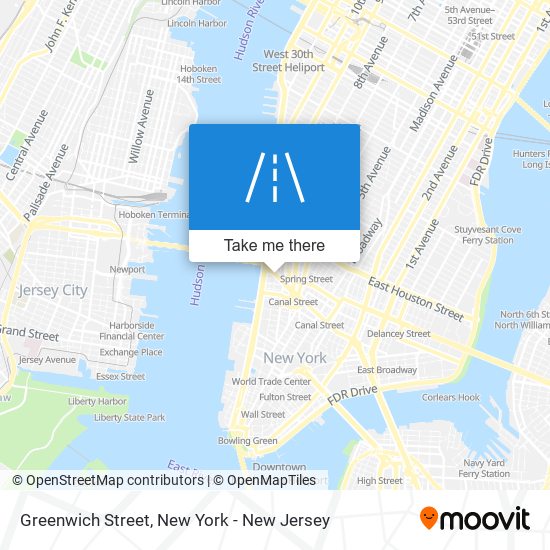This image features an intricate map of New York City, highlighting key landmarks and routes. At the center of the map is Manhattan, bordered by the Hudson River which separates New York from New Jersey. The map prominently shows Canal Street, Spring Street, the World Trade Center, and Fulton Street. 

Major roads are depicted with bold yellow lines, while side streets are marked with finer white lines. At the bottom left corner, there is a copyright notice which reads "© OpenStreetMap Contributors" followed by another mark stating "© OpenMapTiles." Under these, the text "Greenwich Street, New York-New Jersey" is visible.

Adjacent to the text is an orange map pin icon with a smiley face, representing the Move It (M-O-O-V-I-T) logo. The main feature of the map includes an inset photo of typical New York City buildings — tan and brick structures, accompanied by street lights, but with minimal pedestrian activity. The scene is set against a clear, bright blue sky, indicating a sunny day. Below the photo, blue text reads "Take Me There," with an arrow pointing northwest of Spring Street. This inset image resembles a Polaroid photo, complete with a small triangle at the bottom, directing attention to a specific spot on the map.